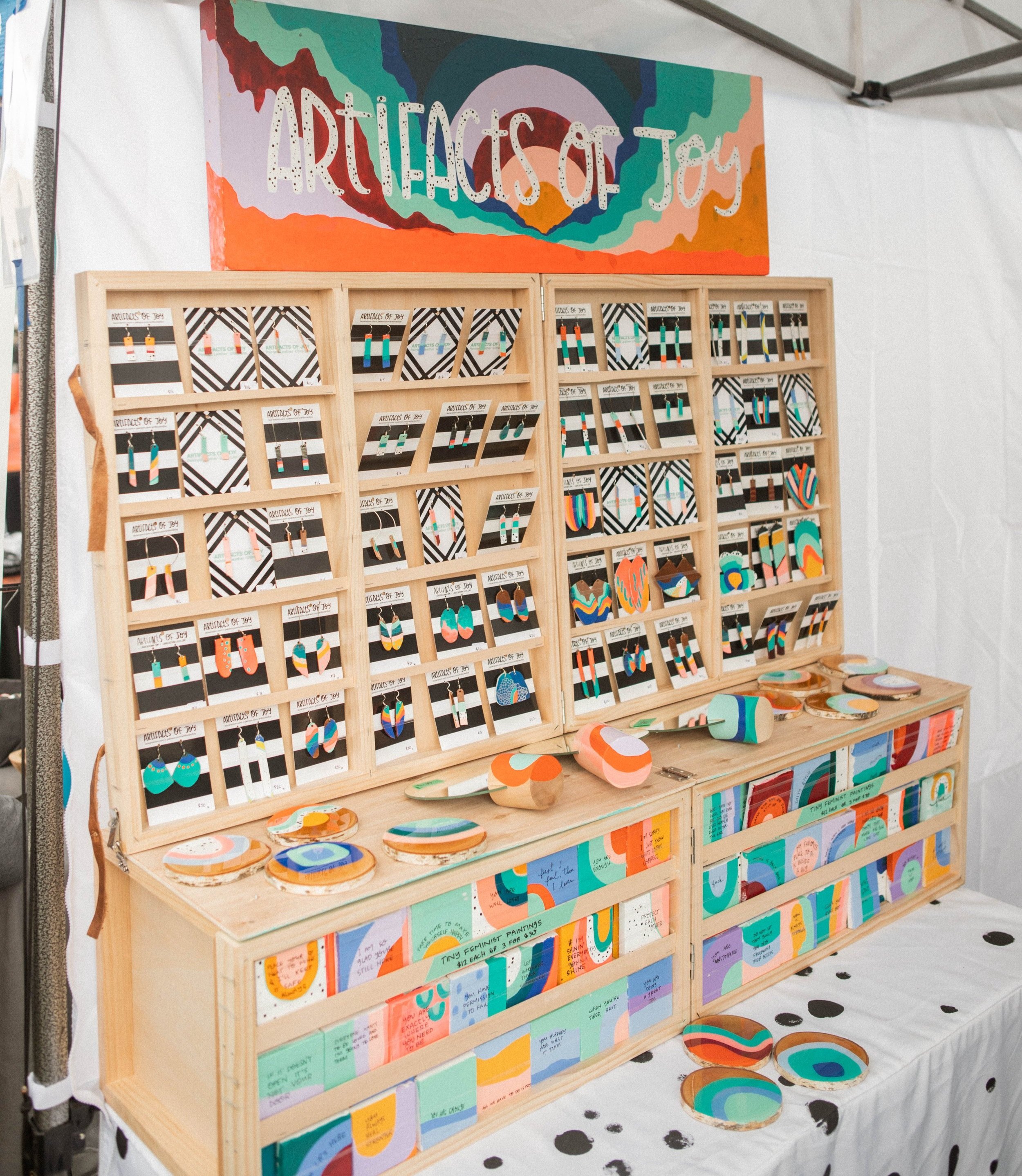The image depicts the inside of a pop-up tent with a white canvas background and visible metal supports. Dominating the center is a display table covered with a white tablecloth adorned with blue or black paint dots. On the table sits an unfinished light-colored wooden chest, highly decorated with bright, pastel-colored squares in shades of purple, mint, blue, and darker blue. These squares, featuring intricate designs and unreadable text, add a vibrant touch to the setup. 

Attached to the back of the chest is a wooden backing, also festooned with decorative elements and pairs of earrings displayed on black and white labels. Above this setup is a rectangular canvas with a colorful sunset in hues of orange, red, blue, and green. In bold white letters with black dots, the sign reads "Artifacts of Joy." The overall ambiance combines the rustic charm of unfinished wood with the bright, pastel-colored details, indicating this could be a booth showcasing handmade jewelry within a bustling market or fair.